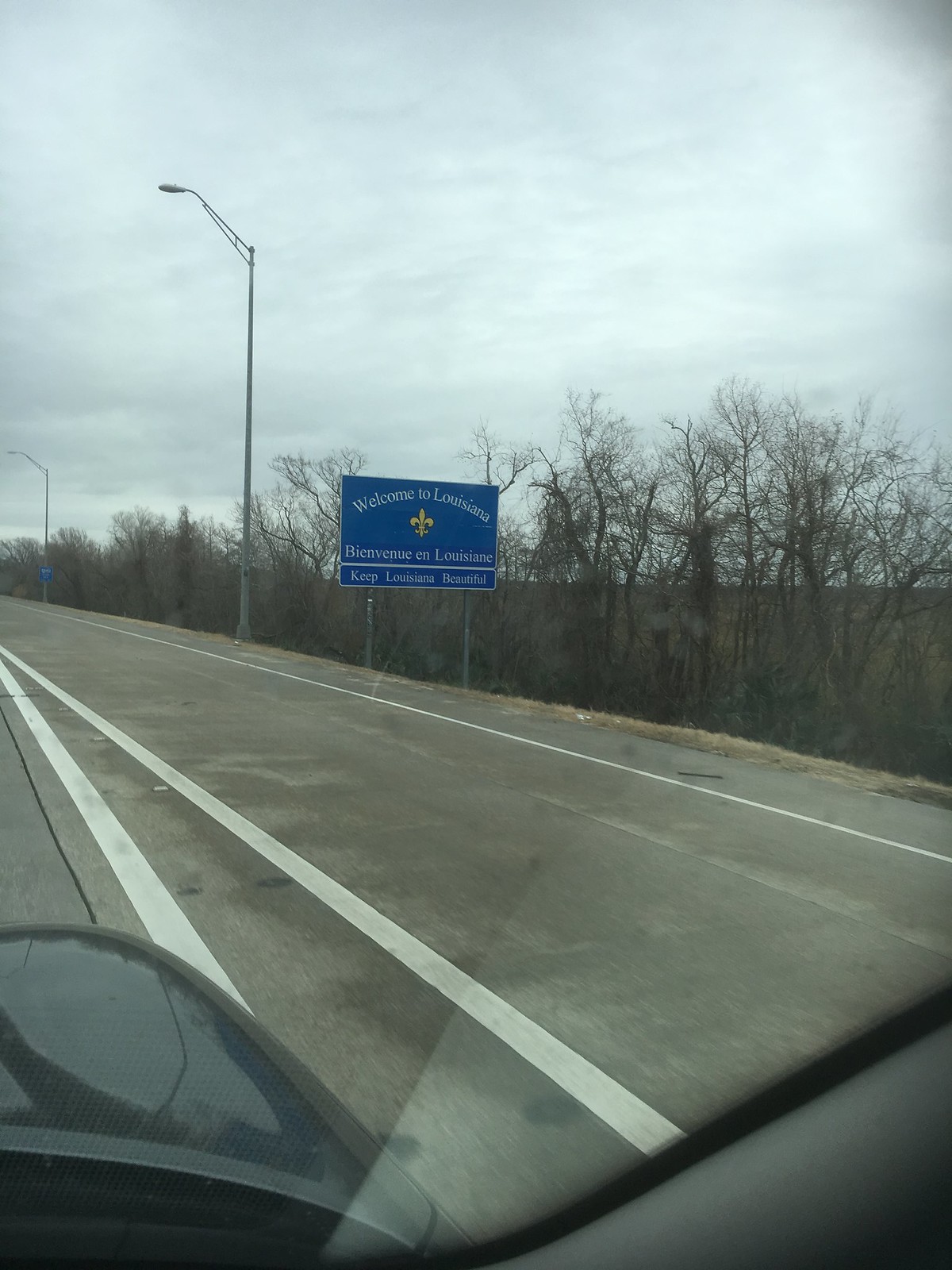In this rectangular image, captured from the perspective of the passenger seat on the right side of a vehicle, we gaze through the windshield at an outdoor scene. The vehicle's interior is dark gray, glimpsed only briefly as the camera primarily focuses on the view outside. The road ahead is gray with a double white line, indicating the vehicle is positioned on the left side, likely on the shoulder.

Prominently, to the right of the road, stands a blue rectangular sign, supported by two silver poles. The navy blue background and white lettering warmly announce, "Welcome to Louisiana. Bienvenue en Louisiane. Keep Louisiana Beautiful." The roadside beyond is lined with numerous trees, bare of leaves, suggesting it is a colder season in Louisiana. The starkness of the trees adds a stark, wintry feel to the welcoming scene.